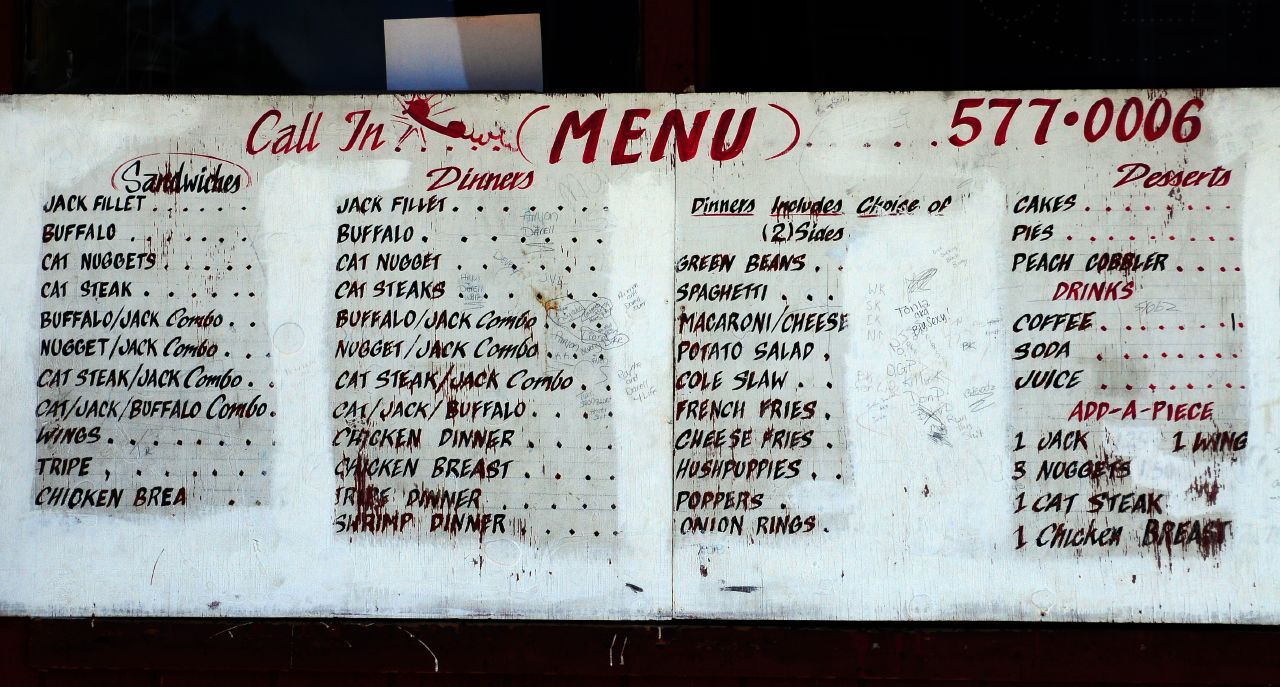At the top of the menu, "Call-In Menu" is prominently displayed in red text. The menu features a white background with a clean layout. In the top left corner, there is a contact number: 577-006. The left side of the menu is dedicated to sandwiches, while the right side lists dinners and desserts.

### Sandwiches (Left Side):
- **Jack Filet**
- **Buffalo**
- **Cat Nuggets**
- **Cat Steak**
- **Buffalo Jack Combo**
- **Nugget Jack Combo**
- **Cat Steak Jack Combo**
- **Cat Jack**
- **Buffalo Combo**
- **Wings**
- **Tripe**
- **Chicken Bray**

### Dinners (Right Side):
The dinners section primarily mirrors the sandwich offerings:
- **Jack Filet**
- **Buffalo**
- **Cat Nuggets**
- **Cat Steak**

Additionally, it includes various side options.

### Desserts (Right Side):
- **Cakes**
- **Pies**
- **Peach Cobbler**

### Beverages:
- **Coffee**
- **Soda**
- **Juice**

The white background provides a neutral canvas that makes the red text and item descriptions stand out clearly for easy readability.